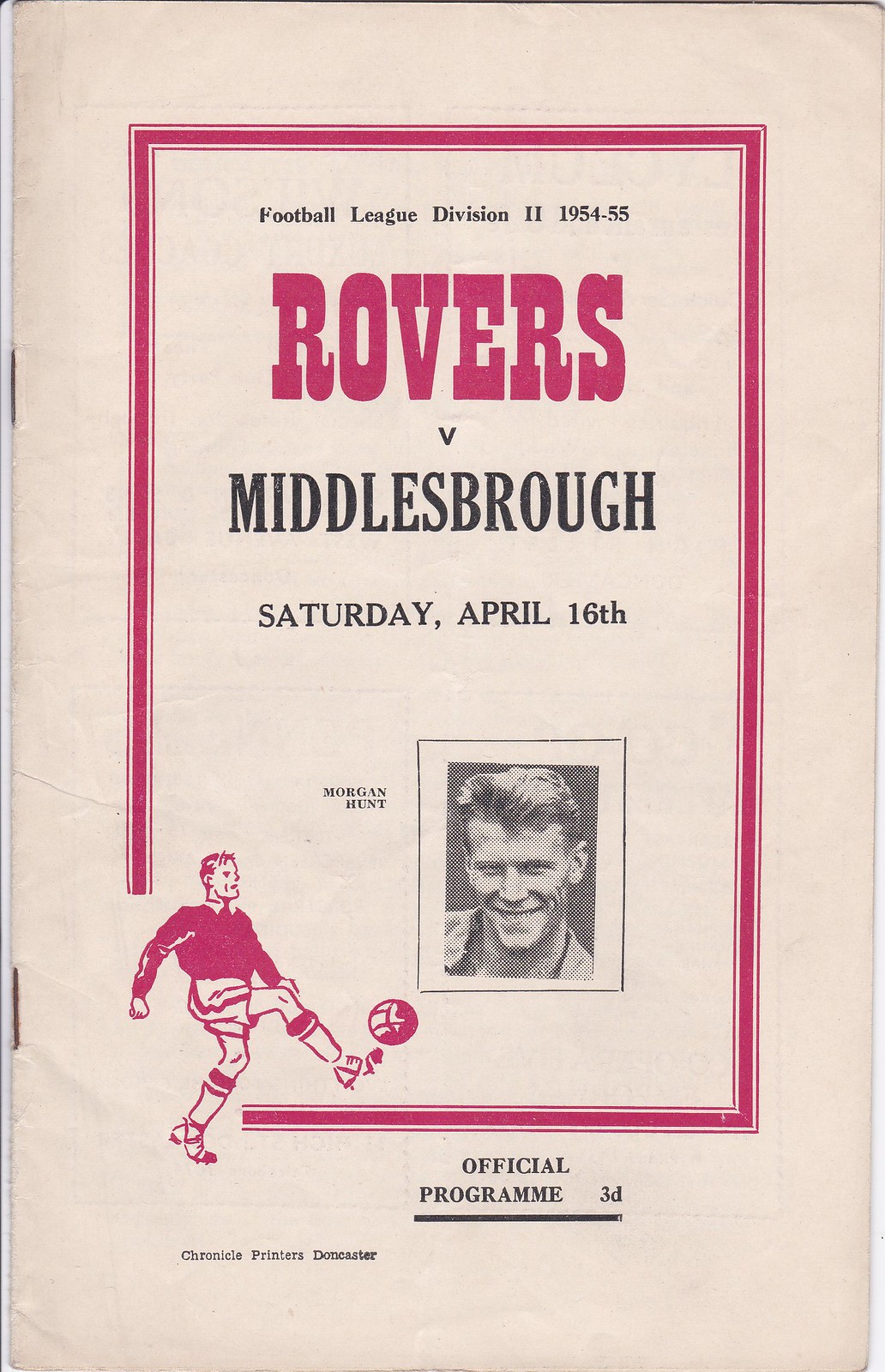The image showcases the front cover of an official program for a soccer match, set against a tannish background. Dominating the center is a maroon-bordered section containing key details. At the top, in bold black text, it reads "Football League, Division II, 1954-55," and just below it, "Rovers vs. Middlesborough, Saturday, April 16th." Central to this maroon-bordered area is a black-and-white portrait of Morgan Hunt, possibly a player. The program uses colors such as tan, black, maroon, and varying shades of gray. Text fills the top and bottom areas, with the main content and the player's picture centrally placed. Additional details include a red-toned, comic-style drawing of a soccer player on the bottom left. At the bottom, in black text, "Official Program 3D" is stated, alongside "Chronicle Printers, Doncaster," indicating the publication and printing details.